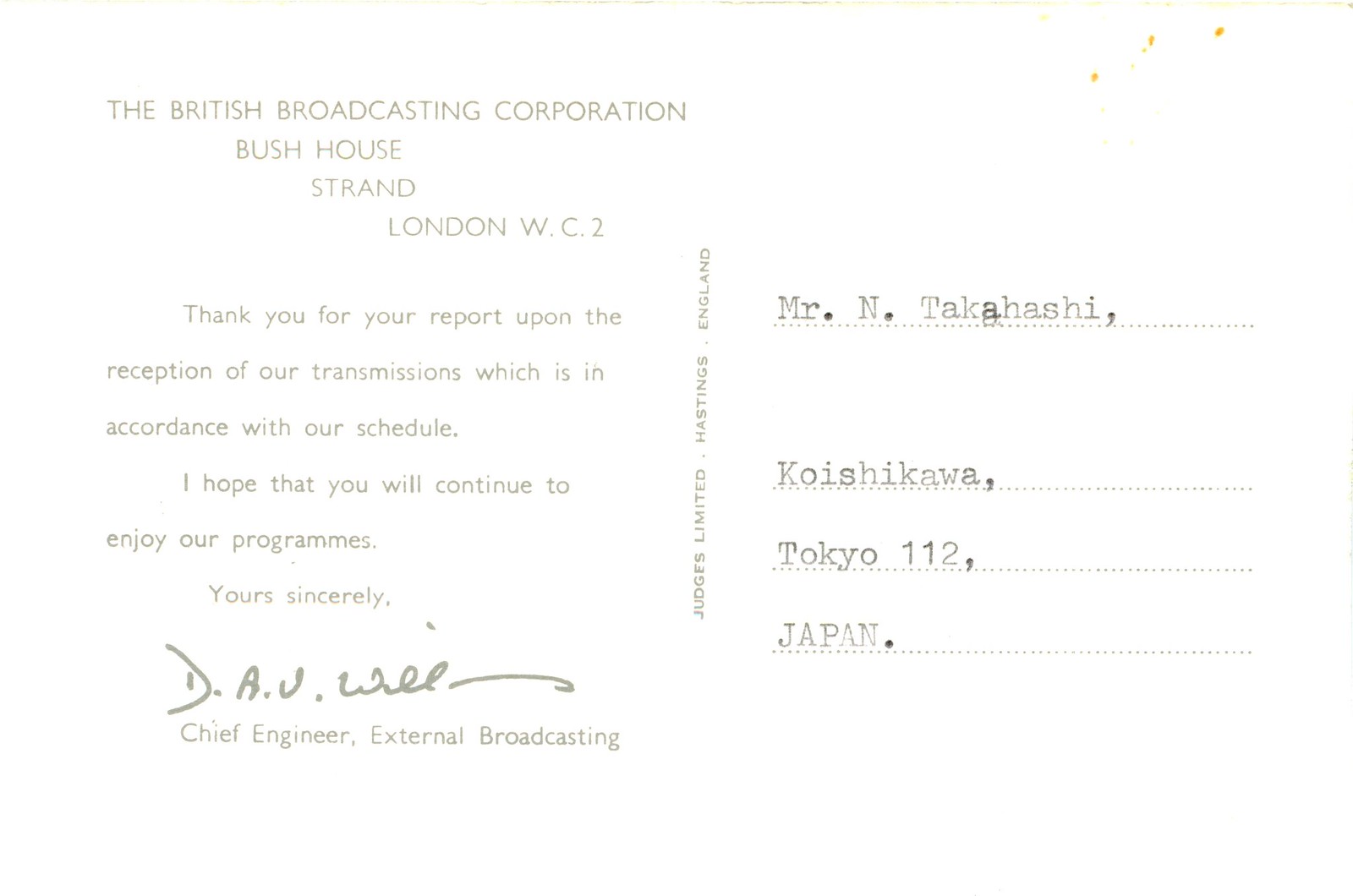This image depicts an old, white postcard with noticeable signs of aging such as faint lines across the top and down the side, and yellow smudges in the upper right-hand corner. On the left side, printed in all-capital black letters, it states the return address: "THE BRITISH BROADCASTING CORPORATION, BUSH HOUSE, STRAND, LONDON, WC2." Below this, there's a message that reads, "Thank you for your report upon reception of our transmissions, which is in accordance with our schedule. I hope that you will continue to enjoy our programs. Yours sincerely, DAV Willis," with a signature followed by the printed title, "Chief Engineer, External Broadcasting." On the right-hand side, the postcard is addressed to "Mr. N. Takahashi, Koishikawa, Tokyo, 112, Japan," with the address neatly typed in, likely via typewriter. Additionally, there are dotted lines indicating the address fields. In the middle of the postcard, there's some text oriented sideways, which reads, "Judges Limited, Hastings, England," further hinting at the era of its origins.